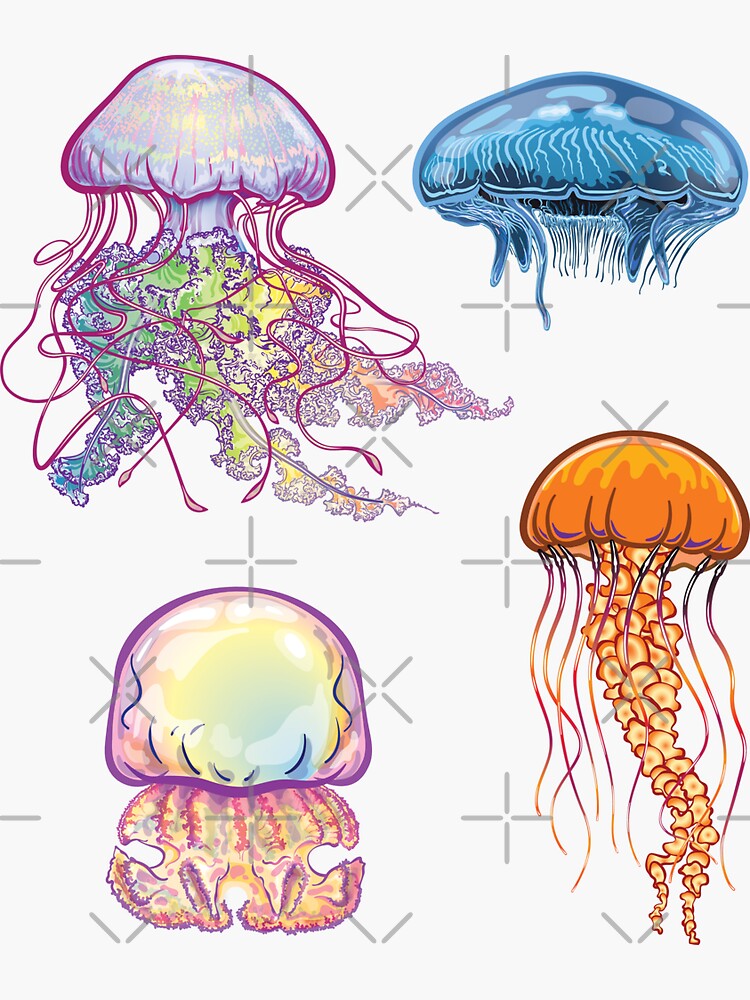This illustration features four distinctively stylized jellyfish rendered in a vibrant array of colors and intricate designs. Positioned in the top left corner, the first jellyfish is a stunning pink specimen with an iridescent sheen and long, ornate rainbow-colored tentacles. This jellyfish displays a combination of purple outlining, light purple filling, and yellow highlighting, with its tentacles featuring a mixture of green, yellow, and coral hues.

The jellyfish in the top right corner is a much shorter blue jellyfish, exhibiting light blue coloring accentuated by a darker blue outline, and it has very short, scarcely visible tentacles, slightly black-tinged underneath. In contrast, the lower right jellyfish is a tall, orange creature with elongated tentacles tinted in orange hues, featuring a central triangular shape that extends downward.

Finally, the bottom left jellyfish is characterized by its shorter structure and a rainbow-colored head, complemented by muted, pinkish rainbow tentacles. Outlined in purple, this jellyfish showcases an interplay of lighter purple, white, yellow, and blue within its margins. All the jellyfish are adorned with little gray pluses and X's on top, adding a unique graphical element to the illustration.